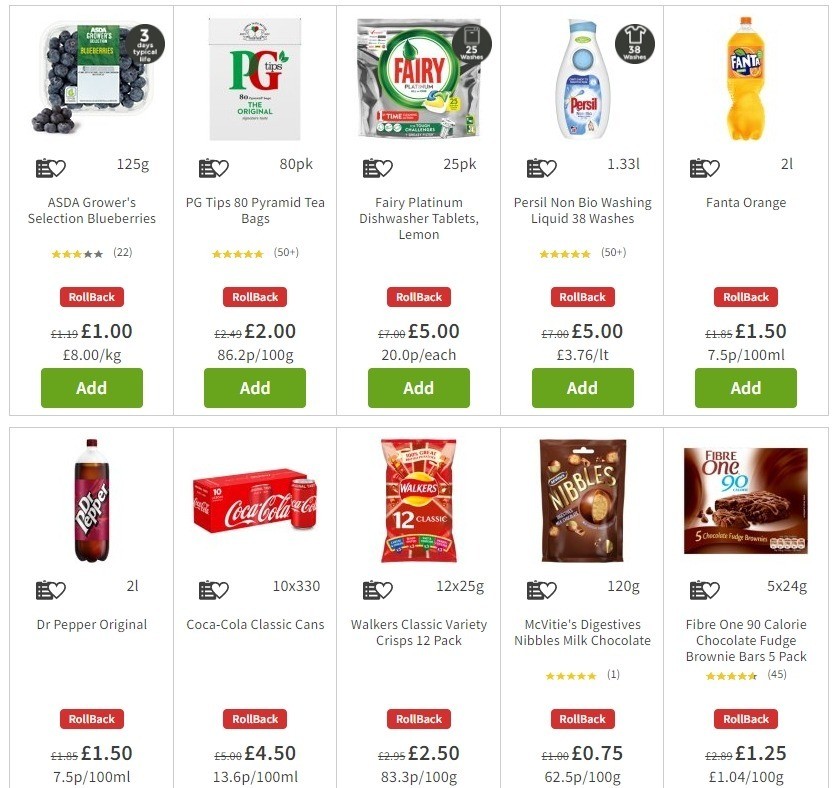The image depicts an online grocery shopping interface for ASDA's Grow Selection. At the top, there are blueberries with a three-star rating from 22 reviews, marked with a red and white "rollback" rectangle, currently priced at one euro. Below, items are listed with similar details:

- **PG Tips AD Pyramid Tea Bags**: Five-star rating with over 50 reviews, priced at two euros, marked with "rollback," and accompanied by a green "add" button.
- **Fairy Platinum Dishwasher Tablets (Lemon)**: Noted with a rollback label, priced at five euros, and also includes an "add" button.
- **Persil Non-Bio Washing Liquid (30 Washes)**: Five-star rating from over 50 reviews, priced at five euros, with a rollback symbol and an "add" button.
- **Fanta Orange Soda**: Marked with a rollback label, priced at one euro and 50 cents, and includes an "add" button.

At the bottom of the list, additional products include:
- Diet Pepsi
- Original Coca-Cola Classic Cans
- Walker's Classic Variety Crisp Multi-Pack
- McVitie's Digestive Nibbles in Milk Chocolate
- 501-90 Calorie Chocolate Fudge Brownie Bars (five pack)

Each item maintains a consistent layout featuring a rollback price, a rating, and a convenient "add" button for easy selection.